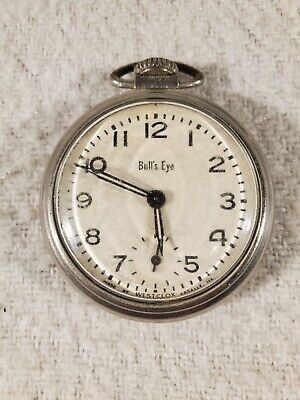This image captures a small, antique pocket watch, distinctly vintage in nature. The watch features a silver casing and a ring at the top for attaching a chain, often worn with a suit. The watch face is white with black numerals and hands, and displays the brand name "Bell’s Eye" by West Clocks at the top. The numbers 1 through 12 are clearly marked, with a notable gap where the '6' should be. Each hour is further divided by small dashes on the clock face. The watch is set to 10 minutes to 6. The background appears to be a soft, gray cloth or paper towel, adding a subtle texture to the setting. Overall, the watch exudes a simple, timeless elegance characteristic of earlier craftsmanship.